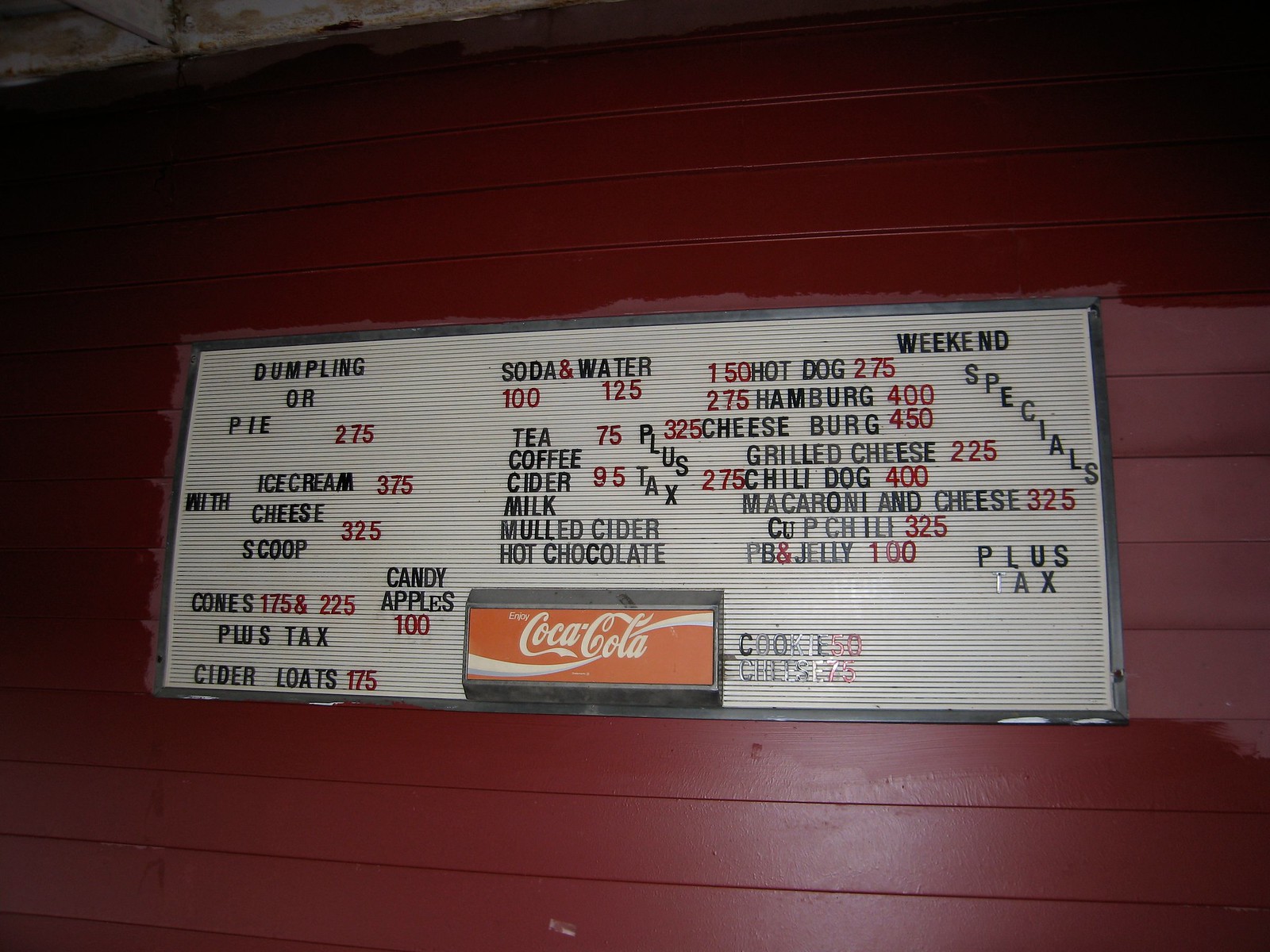This vibrant color photograph captures a vintage-style white menu board mounted on a striking red-painted wall. The board itself is the classic type where individual letters are inserted to display menu items and prices. A prominent red rectangle at the bottom center of the board features the iconic slogan, "Enjoy Coca-Cola," with "Coca-Cola" scripted in its famous trademark font.

The menu starts from the left and lists various items along with their prices. The offerings include:

- Dumpling or Pie: $2.75
- Ice Cream: $3.75
- With Cheese: $3.25
- Scoop Cones: $1.75 and $2.25 plus tax
- Cider Floats (noted humorously as "L-O-A-T-S" due to a missing letter): $1.75
- Candy Apples: $1.00
- Soda and Water: $1.00 and $1.25
- Tea: $0.75
- Coffee, Cider, Milk, Mulled Cider, Hot Chocolate: each $0.95 plus tax
- Hot Dog: $1.50 or $2.75
- Hamburger: $2.75 or $4.00
- Cheeseburger: $3.25 or $4.50
- Grilled Cheese: $2.25
- Chili Dog: $2.75 and $4.00
- Macaroni and Cheese: $3.25
- Cup Chili: $3.25
- PB and Jelly: $1.00
- Weekend Specials (plus tax)
- Cookies: $0.50
- Cheese: $0.75

The words "cookies" and "cheese" are somewhat obscured by a reflection, likely due to a nearby light source, making them harder to read clearly. The menu offers a charming, nostalgic glimpse into a variety of affordable, classic treats and beverages.